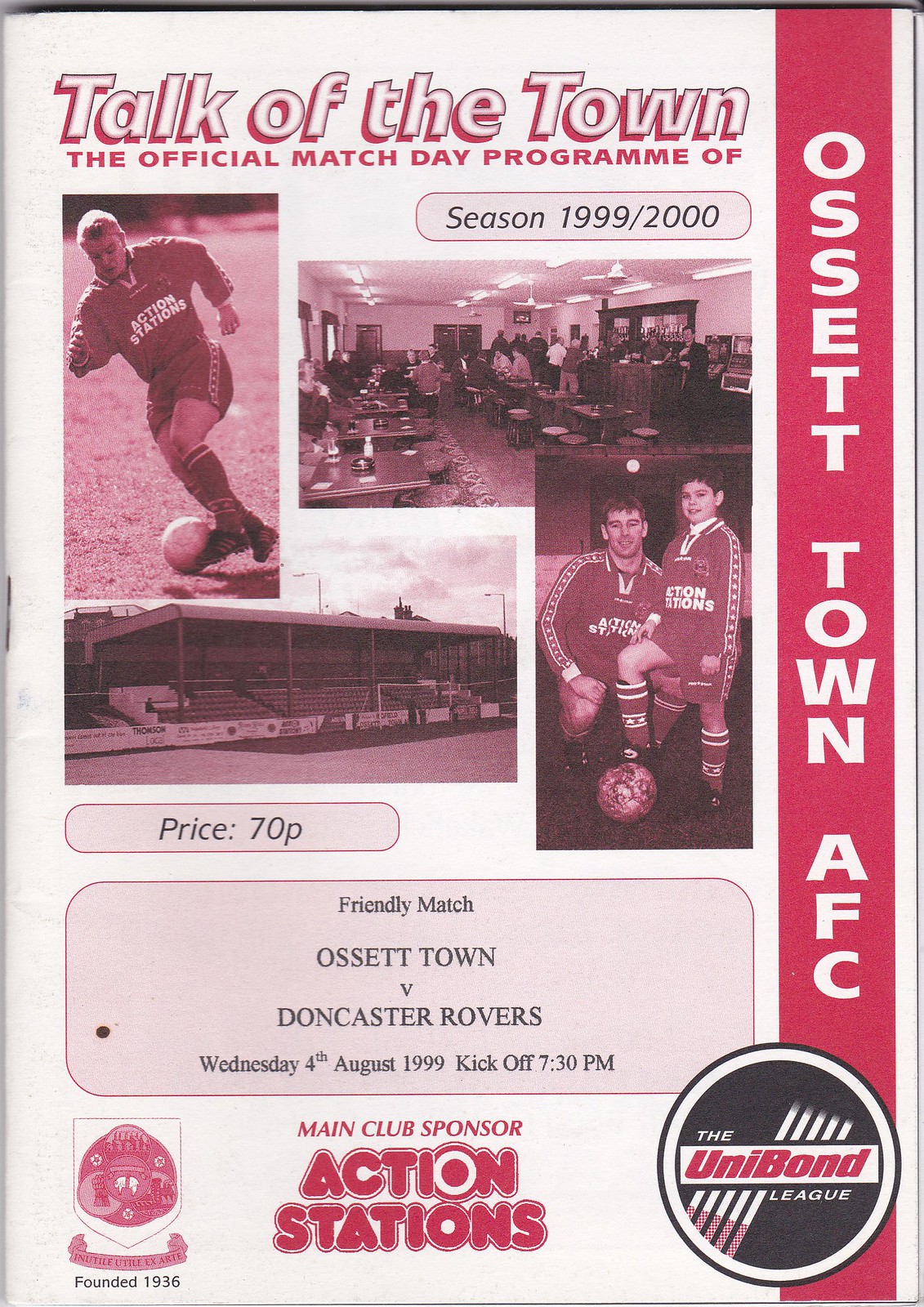The image is the front page of the "Talk of the Town" match day program for Ossett Town AFC's 1999-2000 season, priced at 70 pence. The program highlights a friendly match between Ossett Town and Doncaster Rovers, scheduled for Wednesday, 4th August 1999, with a kick-off at 7:30 pm. Sponsoring the event is Action Stations, prominently featured on the cover. The program is associated with the Unibond League, founded in 1936. The middle of the cover displays four pictures: a man in full soccer attire kicking a ball with "Action Stations" on his shirt, an image of a cafeteria, empty bleachers, and a young child with his right foot on a soccer ball, accompanied by a crouching man.